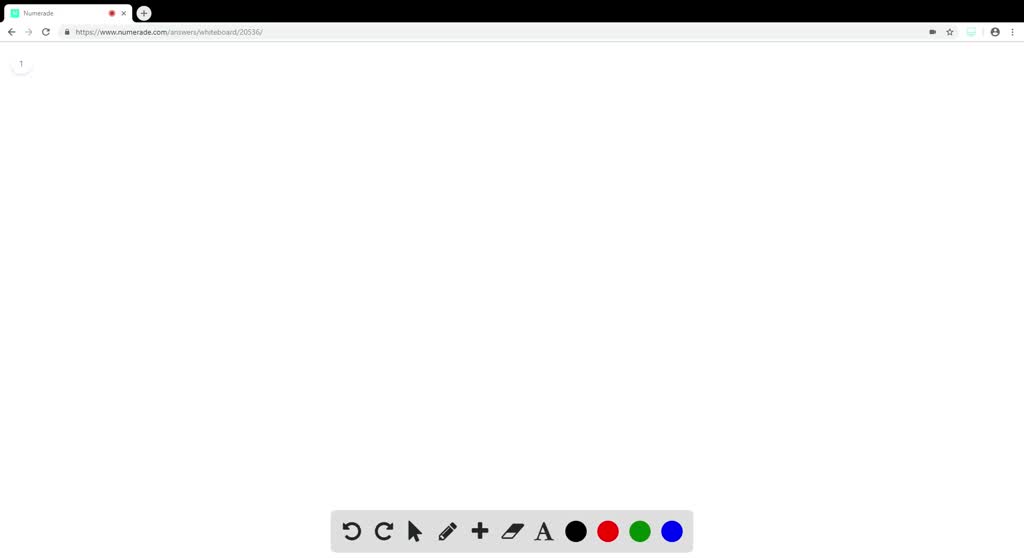Detailed Caption: This image is an incomplete screenshot of a web browser window with a distinct black frame. The browser tab is visible at the top, displaying a teal box logo with an 'M' on it and a numbered label. On the right side of the tab, there are additional icons including a record icon and an 'X' button for closing the tab.

Moving down to the toolbar, it contains several elements: a back button, a forward button, a refresh button, and an address bar. The address bar shows a lock icon next to the URL "numery.com," indicating a secure connection. To the right of the address bar, there is another record icon, a star icon for bookmarking, and a profile icon.

The main body of the webpage itself is largely blank, with just a single element located in the top left corner. Below the blank white space is a gray stripe situated in the bottom center of the screen, containing various icons, hinting at functionality related to drawing or commenting. These icons include back, forward, arrow, pencil, plus, eraser, a text icon (starting with an 'A'), and four color palette options in black, red, green, and violet.

The overall webpage appears minimalistic, with the primary graphical focus on the toolbar and the tool icons at the bottom center.